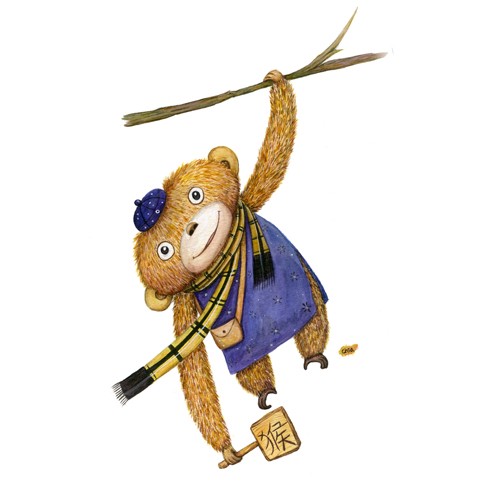In this illustrated image, a cartoon-like character, resembling a bear or potentially a sloth, is depicted hanging from a horizontal, brown branch against a blank white background. The creature has a textured fur and wide head, giving it a whimsical appearance. It clings to the branch with its left arm, while its other limbs dangle freely. The character is adorned with a blue painter's cap (or possibly a yarmulke) and a yellow scarf with blue or black stripes. It wears a blue shirt or tunic, and carries a brown mail carrier bag, resembling an envelope. In its right hand, extended downward, it holds a sign inscribed with Chinese or Japanese characters. There appears to be an indistinguishable object near its feet, possibly an artist's signature or a small item such as a peanut, adding a subtle detail to the composition.